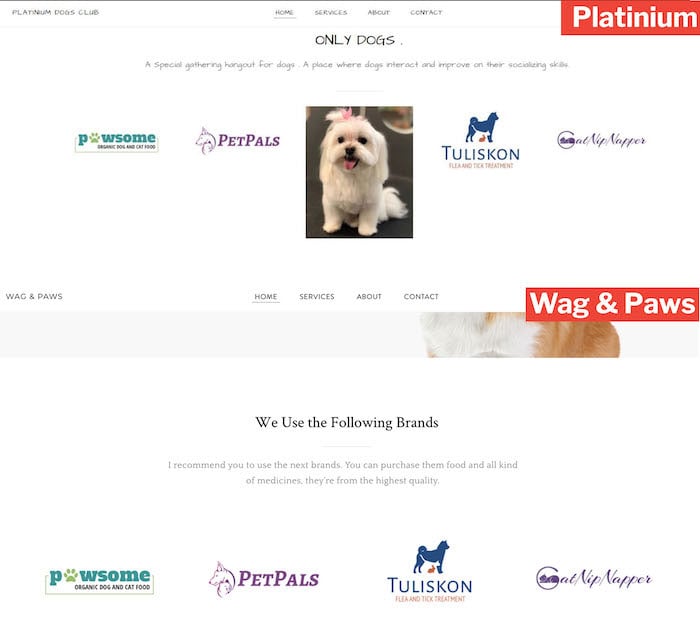In the center of the image, there is a photo of an adorable white Maltese dog, sitting on a dark floor with a pink ribbon adorably tied on the top of its head. Above the dog, text reads, "Only Dogs - A special gathering hangout for dogs. A place where dogs interact and improve on their socializing skills." In the upper left corner of the screenshot, the text "Platinum Dogs Club" is prominently displayed. Across the center of the image, there are navigation options labeled "Home," "Services," "About," and "Contact." In the lower right corner, set against a vibrant red background, white block text reads "Wag and Paws." To the left of this, there are again navigation options: "Home," "Services," "About," and "Contact." At the bottom of the image, spanning from left to right, are logos of various pet-related companies. They include "Pawsome Organic Dog and Cat Food," "Pet Pals," "Taliscon Flea and Tick Treatment," and "Catnip Napper." This detailed composition suggests a professional, pet-centered business interface.